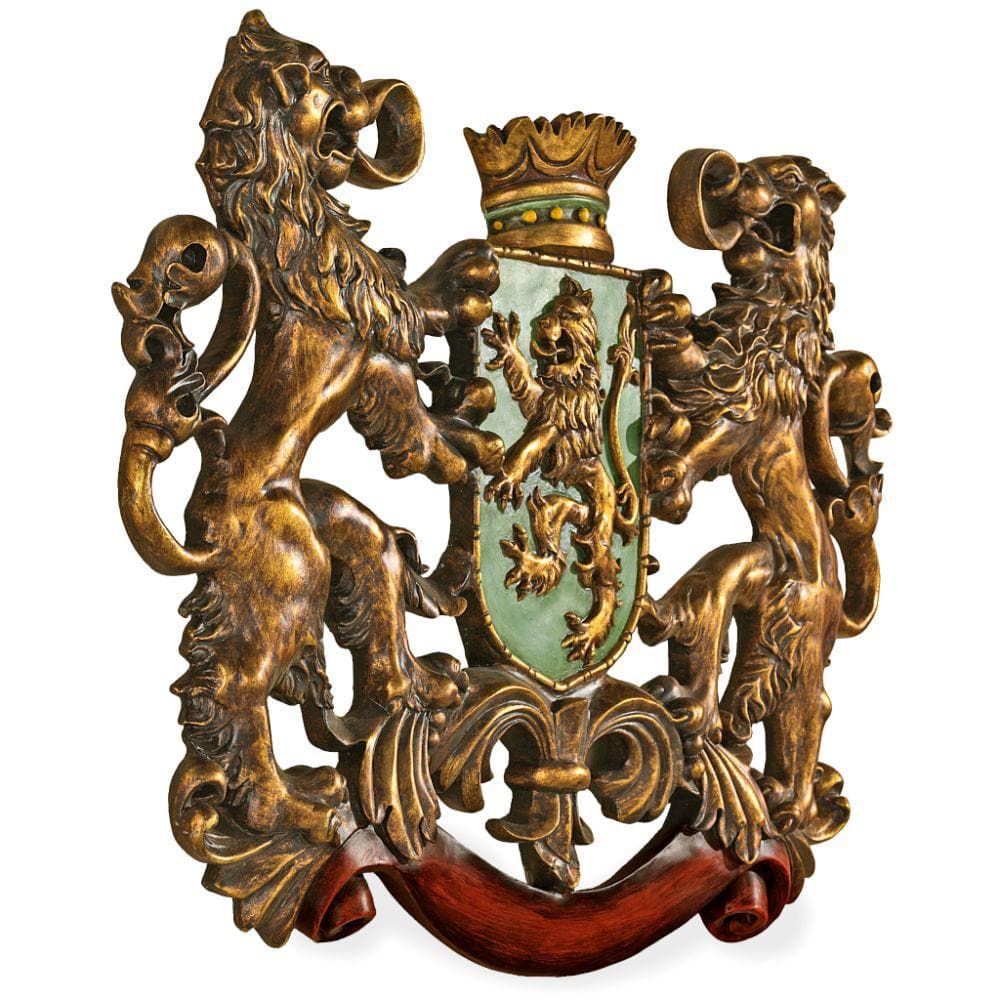This image depicts an intricately carved medieval-style crest, appearing to be made from a single piece of wood. The central elements of the crest include two lions standing on their hind legs, each placed symmetrically on either side of a shield and appearing to support it with their forepaws. Above them, a golden crown sits majestically atop the shield. The shield itself has a green background and houses a detailed gold lion, also standing on its hind legs, with its mouth open, tongue visible, and front claws extended as if lunging to the right. Below the shield, there is a red ribbon, which curves elegantly up at each end and has a glossy finish. The detailed carving includes distinct features such as the lions' manes, faces, eyes, and paws. The entire piece is characterized by a dark golden-brown hue, enhancing its rich, historic appearance.